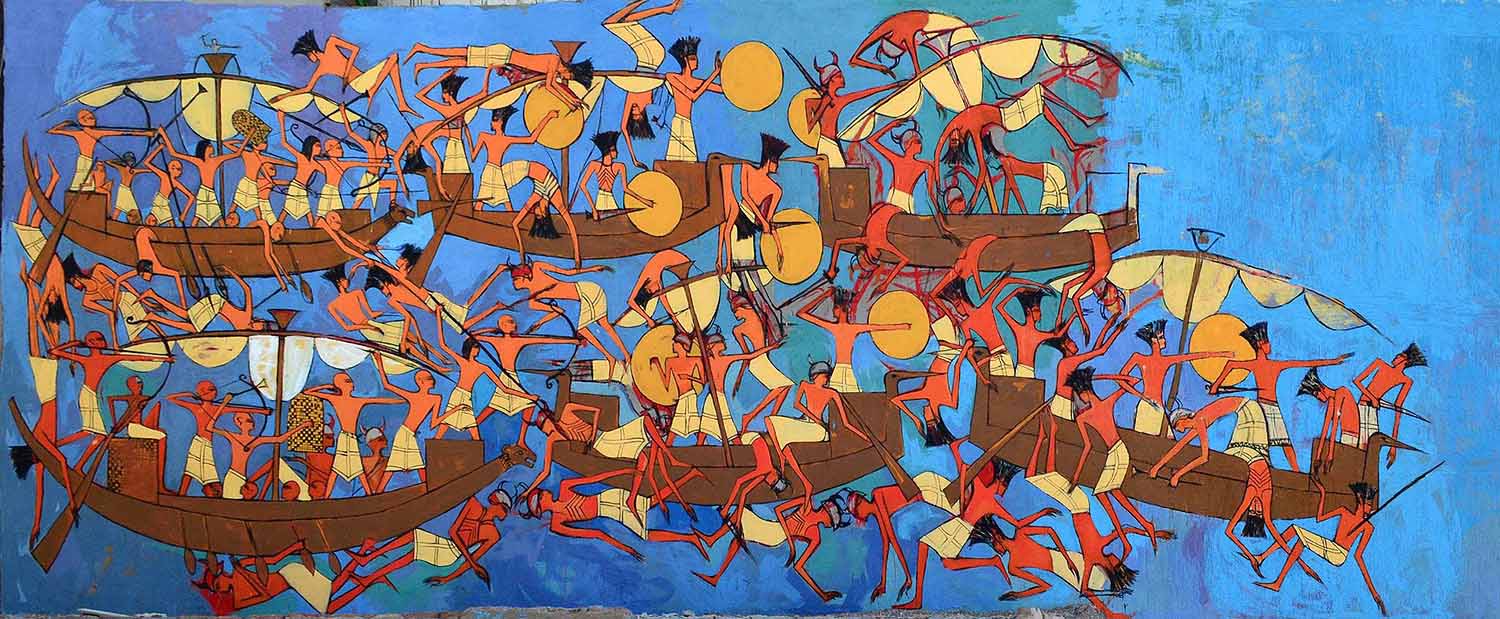This colorful ancient Egyptian painting depicts a chaotic naval battle scene. Spread across six wooden boats, the Egyptians, dressed only in characteristic white skirts adorned with black patterns, are engaged in intense combat. Some wield weapons such as bows, arrows, spears, and swords, while others hold shields. The figures display a range of skin tones, from deep reddish hues to lighter orange and brown. The boats, seemingly stacked atop one another in a slightly abstract manner, travel from the left to the right of the painting. Surrounding the tumultuous scene, some sailors are in the water or shown in various dynamic positions—standing, falling, or seemingly floating above the boats. The background features an electric blue ocean, with varying shades that add depth and intensity to the scene. The characters' distinctive headgear and skirts evoke typical styles found in hieroglyphic depictions of ancient Egyptian life, reinforcing the historical context of this vibrant and intricate artwork.